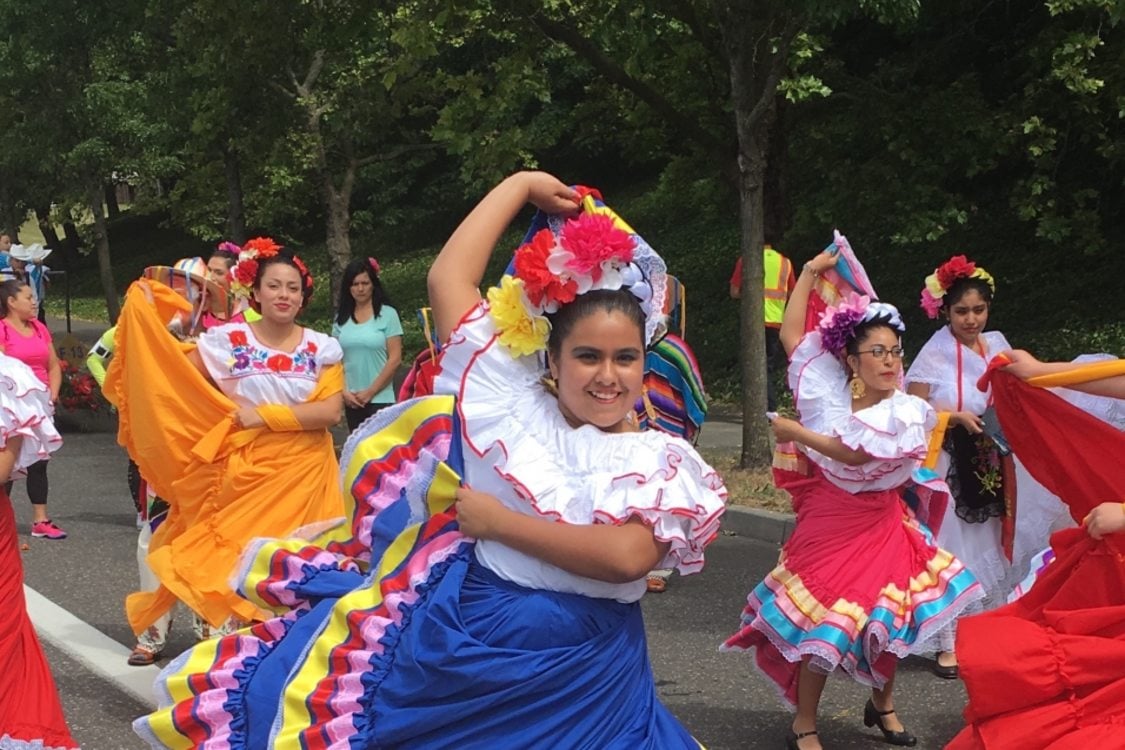This vibrant, professionally taken photograph captures a lively street scene, likely part of a cultural parade or celebration, possibly of Hispanic origin. The foreground is filled with a group of women and children performing a synchronized dance, all wearing traditional attire. The dancers, who are predominantly dark-skinned, exude joy and energy as they engage with the camera and each other. Each woman wears a puffy white blouse adorned with red accents and frilly sleeves, paired with skirts of various colors including orange, blue, pink, and red. The skirts vary in length but generally fall below the knee, with some featuring intricate patterns and stripes at the hem. Complementing their outfits are colorful flower headbands in shades of purple, yellow, red, and pink.

The background of the image shows lush green trees with slender brown trunks, and the dancers move on a gray asphalt road, flanked by a sidewalk. To the center right, a person wearing a yellow safety vest faces away from the camera, while to the center left and far left, additional onlookers in non-traditional attire, such as a pink shirt and teal green t-shirt, can be seen. The scene suggests a sunny or temperate day, adding to the celebratory feel of the moment. The absence of any text in the image focuses attention entirely on the dancers and their colorful, expressive costumes, creating a vivid portrayal of cultural festivity and communal joy.